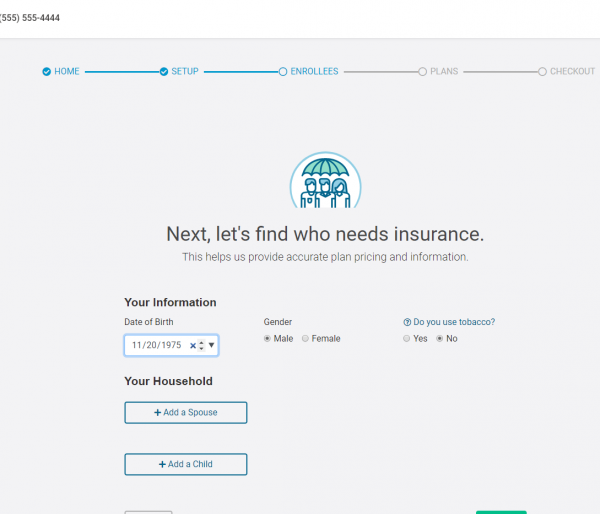This is an image captured from an insurance company's website. At the very top of the webpage, the company's phone number is displayed prominently in black print. The overall background of the website is a subdued gray.

Starting from the upper section, the navigation bar lists several steps. The first step, labeled "Home," is highlighted in blue with a check mark beside it. A connecting blue line leads to the next step, "Setup." Continuing to the right, another blue line progresses to "Enrollees," which does not yet have a check mark. Beyond this, a gray line extends towards "Plans" and another towards "Checkout," indicating future steps that have not been completed.

Below the navigation bar, there is an animated illustration of three people standing under an umbrella, symbolizing protection or coverage. Accompanying this image is the text: "Next, let's find who needs insurance. This helps us provide accurate plan pricing and information."

Following the illustration, a section labeled "Your Information" appears. It includes fields for personal details:
- Date of Birth: Filled in as "11/20/1975" with an option to adjust it via a drop-down menu.
- Gender: Selected as "Male."
- Do you use tobacco?: Selected as "No."

There is also a section titled "Your Household" with options to add additional members: "Add a Spouse" and "Add a Child." The visible portion of the website ends here, indicating that more options and steps follow beyond the current view.